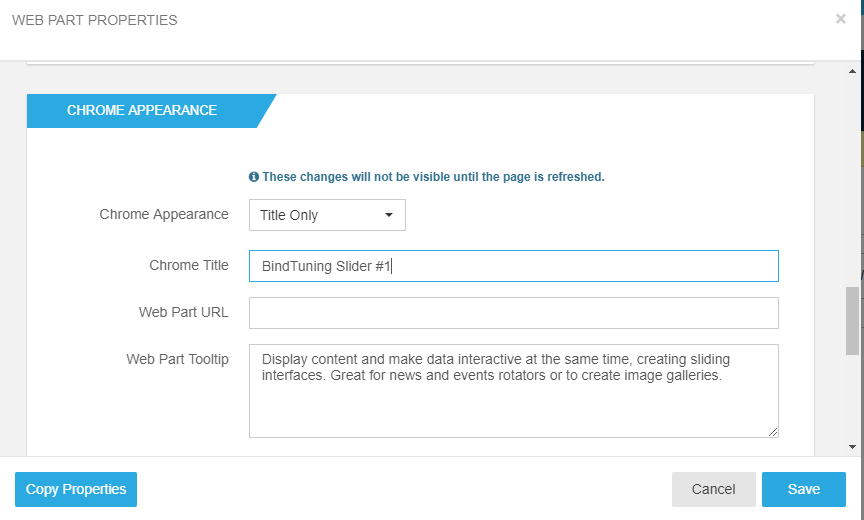The image depicts a user interface layout with two horizontally elongated rectangles, one placed inside the other. The outer rectangle has a gray background, while the inner rectangle, which is also horizontally elongated, features a white background. 

In the upper left corner of the white rectangle, there is a blue section with white text that reads "Chrome appearance." This blue section extends slightly beyond the text.

Below this, centered within the white background, there is an icon consisting of a circle with the letter "I" in the middle. Accompanying this icon, a line of text states: "These changes will not be visible until the page is refreshed."

Further down, on the left side, the text "Chrome appearance" is positioned above a dropdown menu that currently displays the option "Title only."

Below the dropdown, the text "Chrome title" appears above a data input field containing the phrase "fine tuning slider number one," with the cursor placed immediately after the numeral one. This field is highlighted with a blue outline.

Subsequently, another text label reads "Web part URL," placed above an empty data input field.

The final label, "Web part tool tip," is above a populated data field containing the text: "Display content and make data interactive at the same time, creating sliding interfaces, great for news and event rotators or to create image galleries."

At the bottom of the white rectangle, there is a blue button on the left labeled "Copy properties" in white text. On the right side, there are two buttons: a gray button with black text reading "Cancel" and a blue button with white text reading "Save."